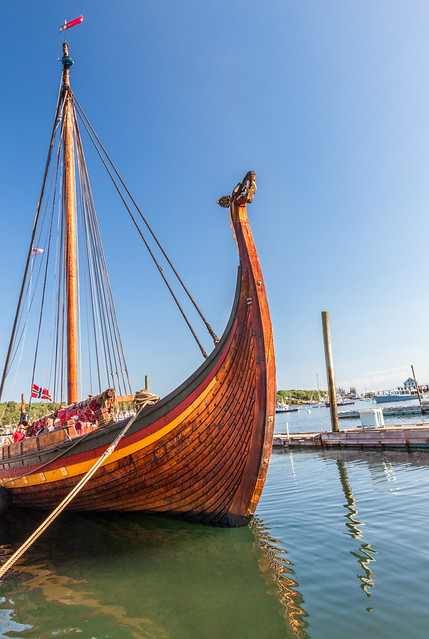This detailed outdoor photographic image depicts the front end of a meticulously crafted wooden replica of a Viking longship, set against a backdrop of clear blue skies and still waters. The ship, exhibiting intricate woodwork with overlapping brown planks, features a carved mythical animal head at the prow, indicating its historical inspiration. The vessel boasts a single tall mast with multiple ropes arranged in a triangular fashion to stabilize it.

Adorning the ship are two prominent flags: a red flag at the top of the mast and a Norwegian flag with a blue cross on a red field at the stern. The boat also has a color scheme along the top edge in red, yellow, and black, reminiscent of the German flag. A rope extends from the side, securing the ship to the shore.

Foreground elements include a visible docking area to the right with a walkway, a pole, and a reflection of these structures in the calm water. The background includes more docks, additional boats, buildings, and trees, enhancing the setting's authenticity. The image captures the ship partially, focusing on its left side and revealing that despite its historical design, it is currently moored, reinforcing its stationary state with reflections visible both under the boat and the dock structures.